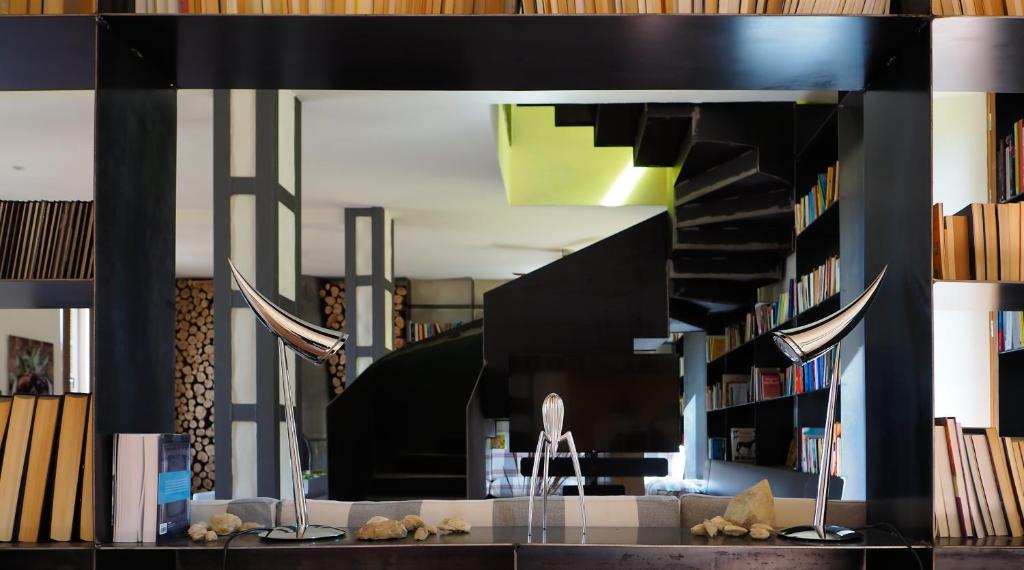The image captures an intricate library scene dominated by a spiraling black staircase at its center, curling upwards towards the upper floor. The foreground features a black countertop adorned with two horn-shaped desk lamps and scattered rocks, with a single book noticeably placed on the left side. The library is framed, possibly through a shelf or mirror, adding a layer of depth. To the sides, multiple levels of bookshelves are lined with books, suggesting an extensive collection, though the titles are indistinguishable due to the distance. The background wall is uniquely constructed with stacks of cut logs neatly filling rectangular spaces, adding a rustic texture to the setting. Some sections of the image appear distorted, contributing to an unusual, almost surreal aesthetic.